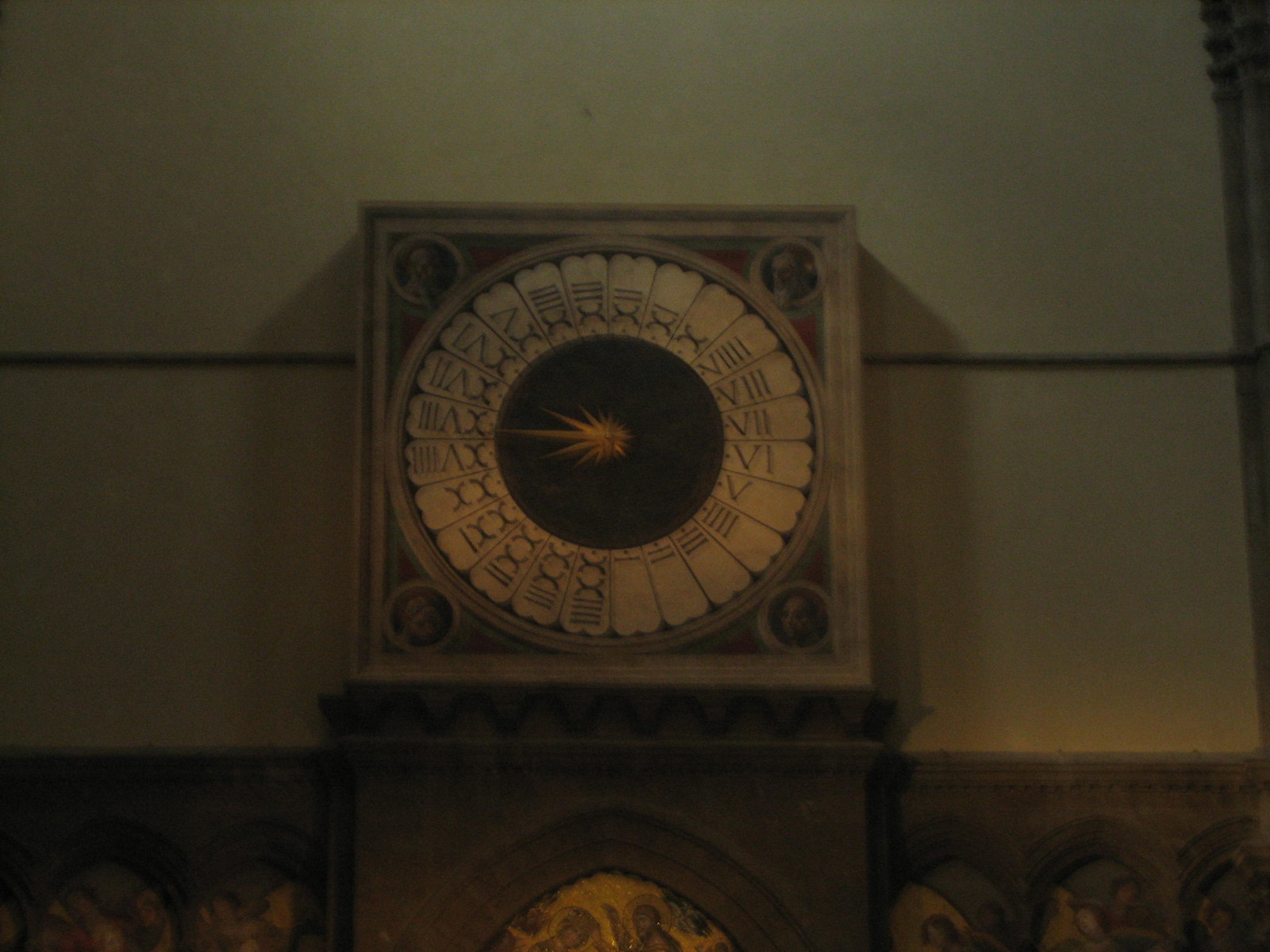A beautifully detailed image captures an antique clock mounted on a wall. The clock, crafted from light wood, features a square face adorned with Roman numerals extending beyond the traditional I through XII, possibly indicating a 24-hour format. At its center, a gold starburst design enhances the elegance of the timepiece. Each corner of the clock is embellished with circular medallions, each portraying the image of a man. The clock's face is marked by a striking black center. Below the clock, an ornately carved wooden platform is positioned, supporting a series of stained glass panels that depict vibrant, artistic scenes from the Bible. The overall aesthetic of the clock and its surrounding elements suggests it is a cherished relic from a bygone era.